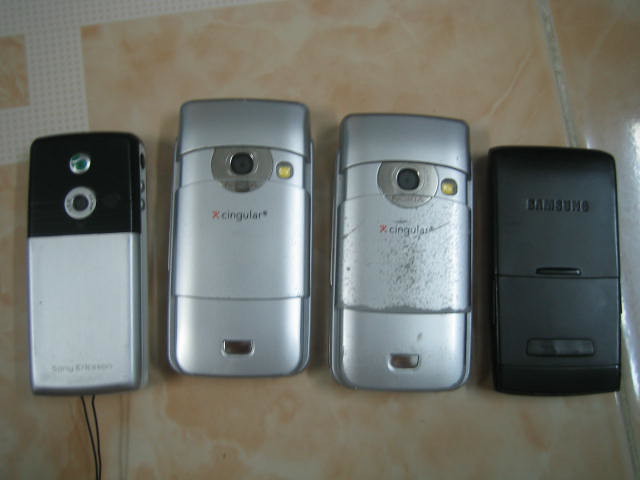This photo showcases four vintage flip phones arranged on a tile floor with a light sheen visible on the right side. The floor resembles white marble laminate with some white textured tape placed on its surface. The phone on the far left is a rectangular, silver Sony model with black accents around the camera, and two thin black wires emerging from its bottom. The two phones in the middle are identical Cingular models, both showing signs of wear with scratches and camera lenses at the top. The phone on the far right is an all-black Samsung flip phone, also marked with signs of use, featuring the Samsung logo prominently at the top.